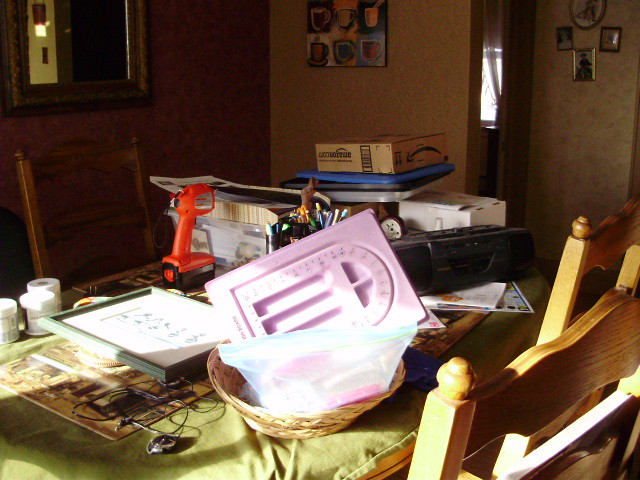The image showcases a cozy, albeit cluttered, kitchen with rustic charm. Dominating the center of the room is a wooden table surrounded by three matching chairs. The table is strewn with a variety of items: an empty Amazon box, a red drill, several placemats, containers of vitamins, a framed piece of art, and possibly a laptop with visible wires. Additionally, a wicker basket contains an unknown item in a lilac hue, while an old boombox with a cassette and CD player brings a nostalgic touch.

Bright light floods in from a window on the left, casting an illuminating glow across the scene. The walls, adorned in dark wallpaper, add a dramatic contrast to the room. In the background, a collection of four vintage photographs hangs on one wall, an art piece graces another, and a mirror is positioned on a third wall, reflecting parts of the room.

In the far end of the kitchen, a doorway reveals a glimpse into a small bedroom, complete with a window and a curtain. The entire scene is devoid of any people and legible text, focusing solely on the potential stories hinted at by the eclectic assortment of objects.